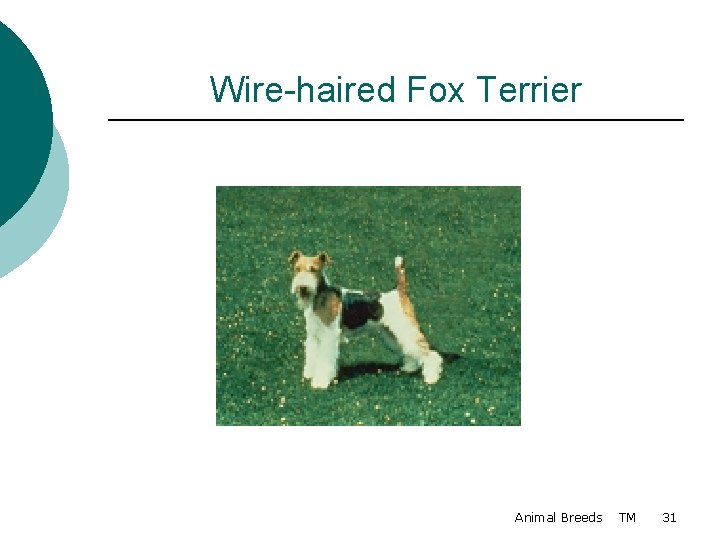The image is likely a poster or placard for a dog breed, possibly featured in a book or at a dog show. This rectangular image prominently displays a wire-haired fox terrier. At the top, in dark green text, it states "Wire-haired Fox Terrier," with a black line directly beneath it spanning from left to right. The dog, situated in the middle, stands proudly in a green field adorned with small yellow flowers, likely dandelions. This multicolored dog is mostly white with light brown and black patches throughout its body. The dog's body faces left while its head looks directly at the camera, showcasing its white snout, white feet, and distinctive brown and black markings on its midsection, shoulders, tail, and head. To the upper left, two half-circle shapes—one in dark green, the other in a lighter bluish-green—add decorative elements to the design. At the bottom right corner, in small black text, is the label "Animal Breeds TM31."